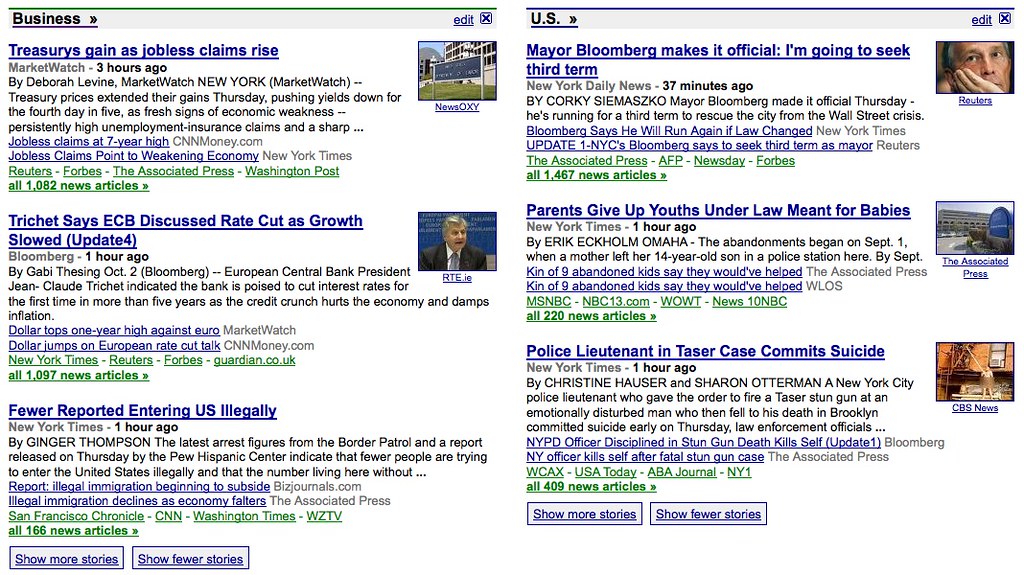In this detailed image, we observe two web search pages displaying a series of news headlines. On the first page, the headlines read: "Business Treasuries Gain as Jobless Claims Increase," reported by MarketWatch three hours ago, and "Trichet Says ECB Discussed Rate Cuts as Growth Slowed [Update 4]." Another headline details, "Dollar Tops One-Year High Against Euro," with an additional snippet stating, "Dollar Jumps on European Rates Court Talk." There is a report from the New York Times, titled "Fewer Reportedly Entering U.S. Illegally," posted one hour ago under the U.S. section. Another notable headline announces, "Mayor Bloomberg Makes It Official: I'm Going to Seek Third Term." Additionally, there's a somber headline stating, "Police Lieutenant in Cesar Case Commits Suicide," published by the New York Times one hour ago. 

On the second search page, similar content is visible with the options to "See More Samples" or "Show Fewer Stories." Another grim update includes "NYPD Officer Disciplined in Stone Gun Death Kills Self," coupled with a parallel headline reading, "New York Officer Kills Self After Fatal Stone Gun Case." 

The image is a reflection of the current news landscape, highlighting significant developments in economics, public policy, legal matters, and tragic events involving law enforcement officers.